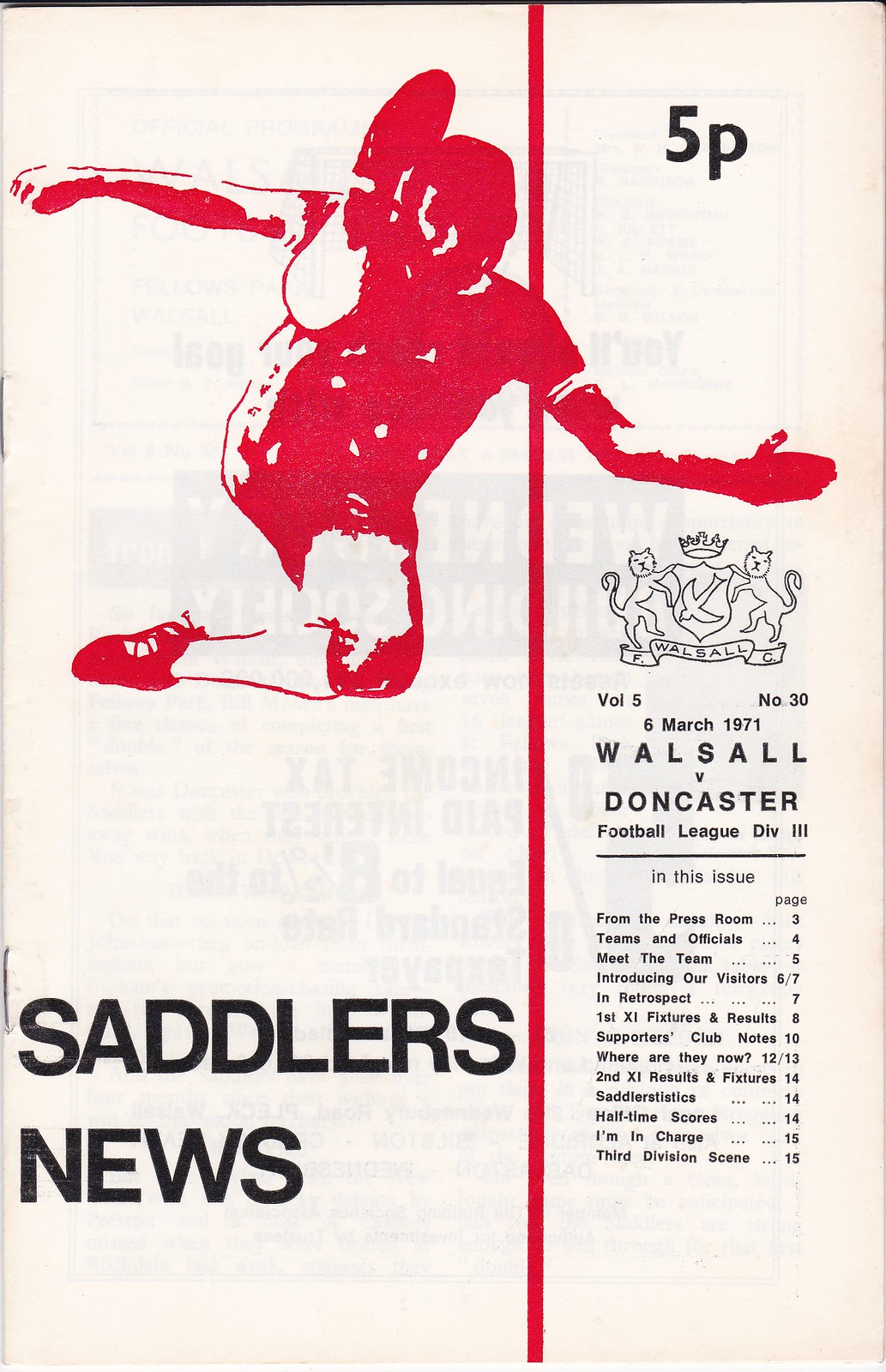The image is a detailed poster resembling an old magazine cover titled "Saddler's News." The background is predominantly white with a pinkish hue. The central focus is a large, red, sketch-style illustration of a football player in mid-air, executing a kick. The player's arms are outstretched to the sides, with the right leg extended forward revealing the bottom of the shoe, and the left leg tucked behind.

In bold black text, the number "5" is visible, from which the letter "P" emerges, indicating a price of "5p." Across the image, additional text reads "Volume 5, Number 30," next to "6 March 1971," and a logo—resembling a family crest with lions—is positioned above. The poster highlights the match "Walsall vs. Doncaster, Football League, Division 3."

The left-hand side of the page is secured together with visible staples, hinting at the handcrafted nature of the magazine. Furthermore, a table of contents is included, stating "In This Issue" with specific mention of "From the Press Room" on page 3, alongside sections such as teams and officials, meet the team, in retrospect, halftime scores, I'm in charge, and third division scene spanning pages 3 through 15.